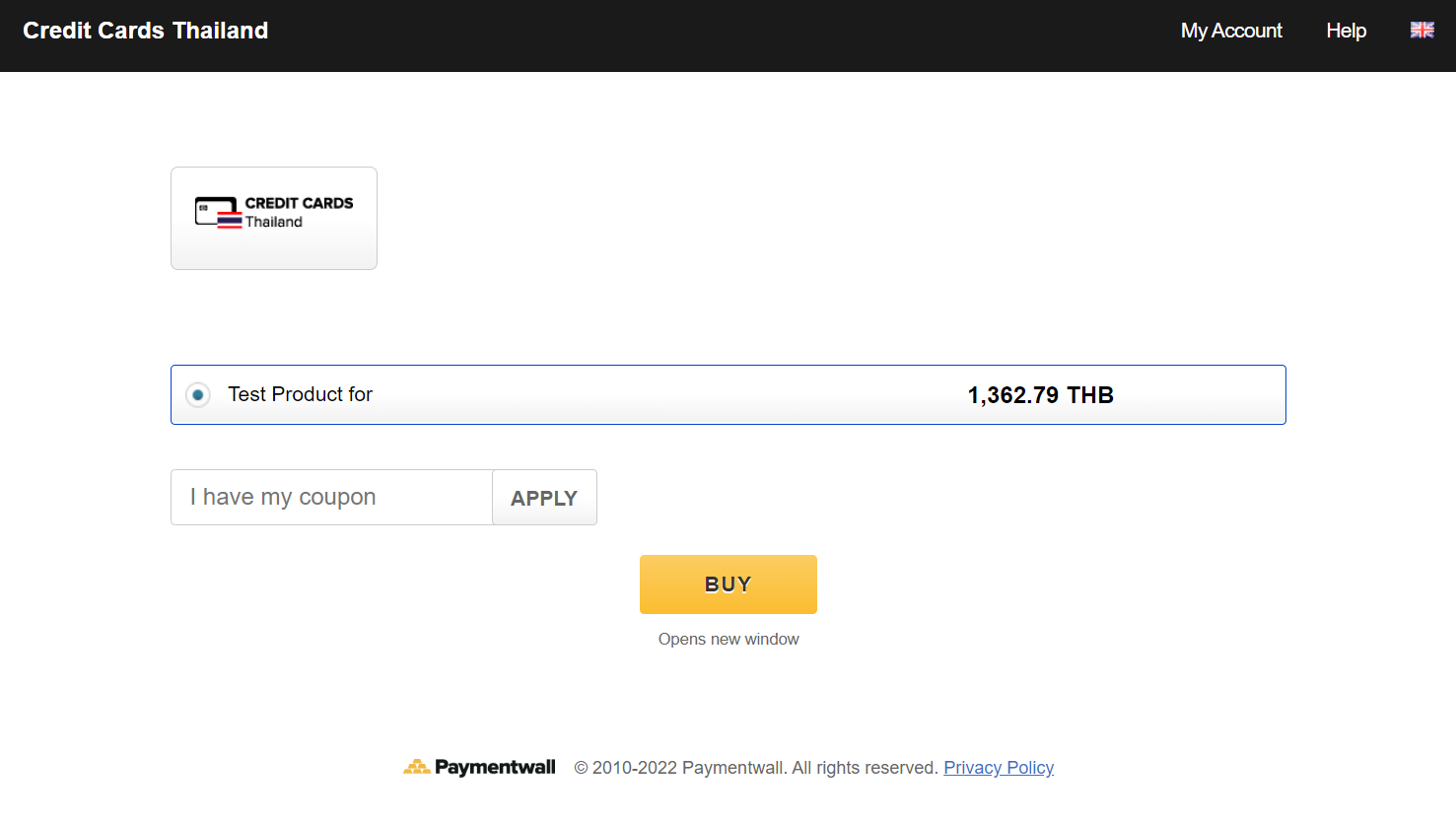Sure, here's a cleaned up and detailed caption for the image:

---

The screenshot displays a web page titled "Credit Cards Thailand" on the top left, showcased on a black background with white text. To the right, the page features options including "My Account," "Help," and a British flag icon. Below the header, the "Credit Cards Thailand" title stands out on a predominantly white background, accompanied by an illustration of the Thai flag featuring red, white, navy blue, white, and red stripes.

The page highlights a selected radio button next to the text "Test Product 4" priced at 1,362.79 Thai Baht, enclosed in a slim bluish rectangle. A section beneath this allows users to enter a promotional coupon code with an "Apply" button next to it. Further down, a large yellow "Buy" button is situated in the lower middle portion of the page. Underneath this button, a note indicates that clicking it will open a new window.

At the very bottom of the page, there is a "Paymentwall" trademark and a timestamp ranging from 2010 to 2022, along with a clickable "Privacy Policy" link.

---

This caption provides a thorough and organized description of the elements present in the screenshot.